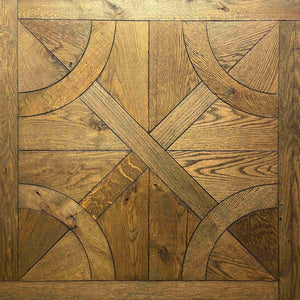This image is a highly detailed, color photograph of a square wooden panel, possibly a flooring tile or tabletop, captured from a top-down perspective. The center of the panel features an intricately designed X shape formed by intersecting wooden pieces. Surrounding the central X, the panel is divided into four distinct sections, each bordered by additional wooden framing. The wood grains vary noticeably in color, showcasing a gradient from light to dark shades. The grains are also oriented in different directions, enhancing the visual complexity of the design. At each corner of the four sections, the wood curves outward in semi-circles, adding to the artistic flair of the panel. The outermost edges are also framed by a border of wood, creating a cohesive and meticulously crafted square structure made up of diverse wooden shapes and cuts.